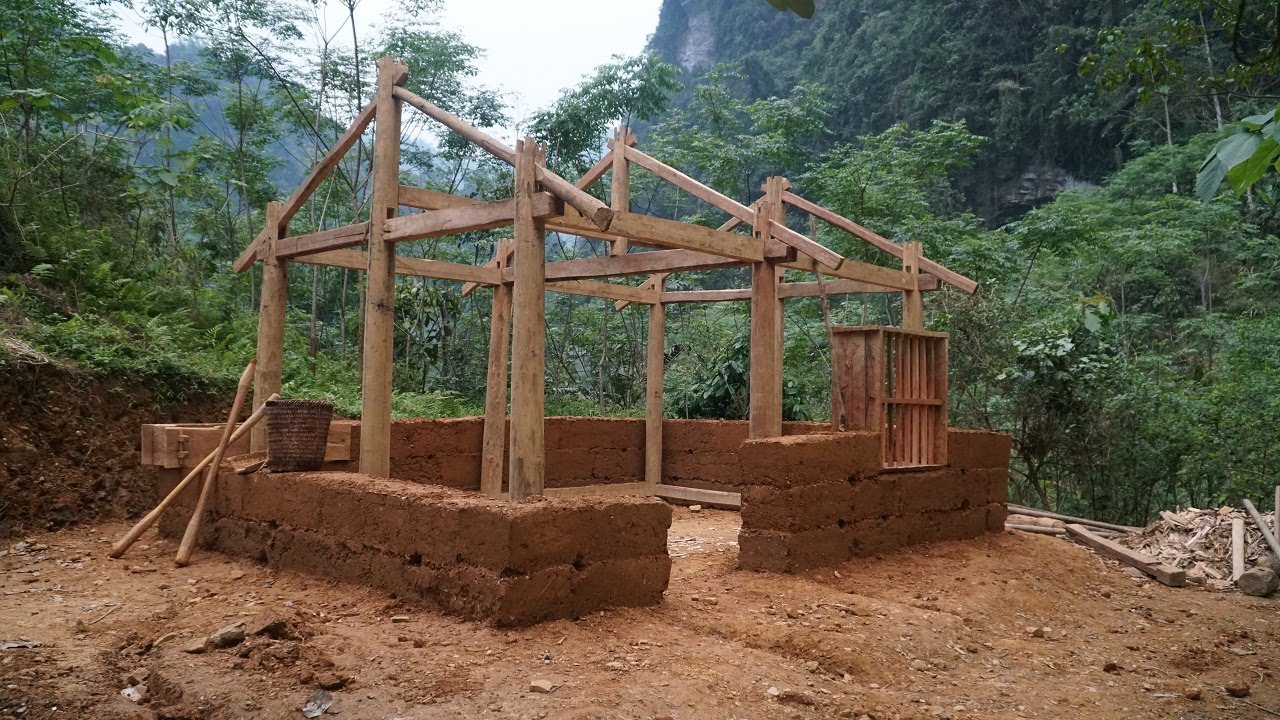This photograph captures the skeletal structure of a hut under construction in the midst of a verdant rainforest. Central to the image is a basic wooden framework set upon a solid foundation of large mud bricks, each approximately two to three feet long and a foot and a half high. The hut features an A-frame roof structure, comprising three triangular formations in a row, with a doorway frame prominently visible but no siding yet affixed. Various tools, including some wooden implements and a metal bucket, lean against the structure, while woven baskets and wood chippings are scattered around the site. The clearing is a mix of brown dirt and stones, with piles of wooden debris on the right. Surrounding the hut, tall, thin trees with lush green foliage frame the background, which also includes the steep slopes of jungle-covered mountains. Although the image is somewhat dark, natural daylight filters through, casting a subtle brightness on the scene.